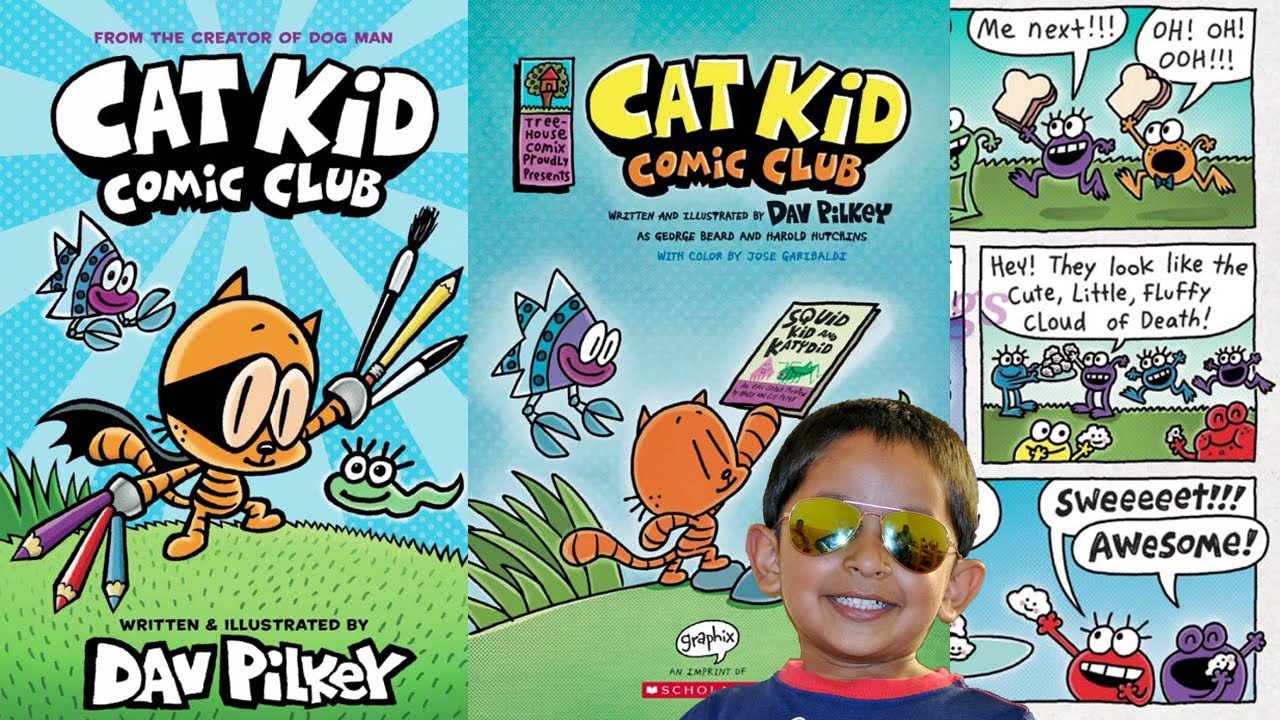Here’s a clean and detailed caption based on the given image description:

"The image features the cover of 'Cat Kid Comic Club' on the left side. The cover is predominantly purple, with the title 'Cat Kid Comic Club' written in large, white letters outlined in black. A note at the top states, 'From the Creator of Dog Man,' in black type. The author credit reads, 'Written and Illustrated by Dav Pilkey' in white letters outlined in black. Depicted on the cover is an orange cat wielding a sword, which is actually a bunch of colored pencils in purple, red, and light blue, standing on a patch of green grass.

In the middle section, another image displays the title 'Cat Kid Comic Club' again but in yellow and orange colors. Here, it also credits 'Written and Illustrated by Dav Pilkey, George Beard and Harold Hutchins, with color by Jose Garibaldi.' The image further depicts a comic with colorful panels and characters. In one of the panels, the words 'Me Next' and 'Oh, Oh' are visible, inside speech bubbles next to characters resembling small, circular creatures. One creature is purple, another is orange, and one is holding a piece of bread."